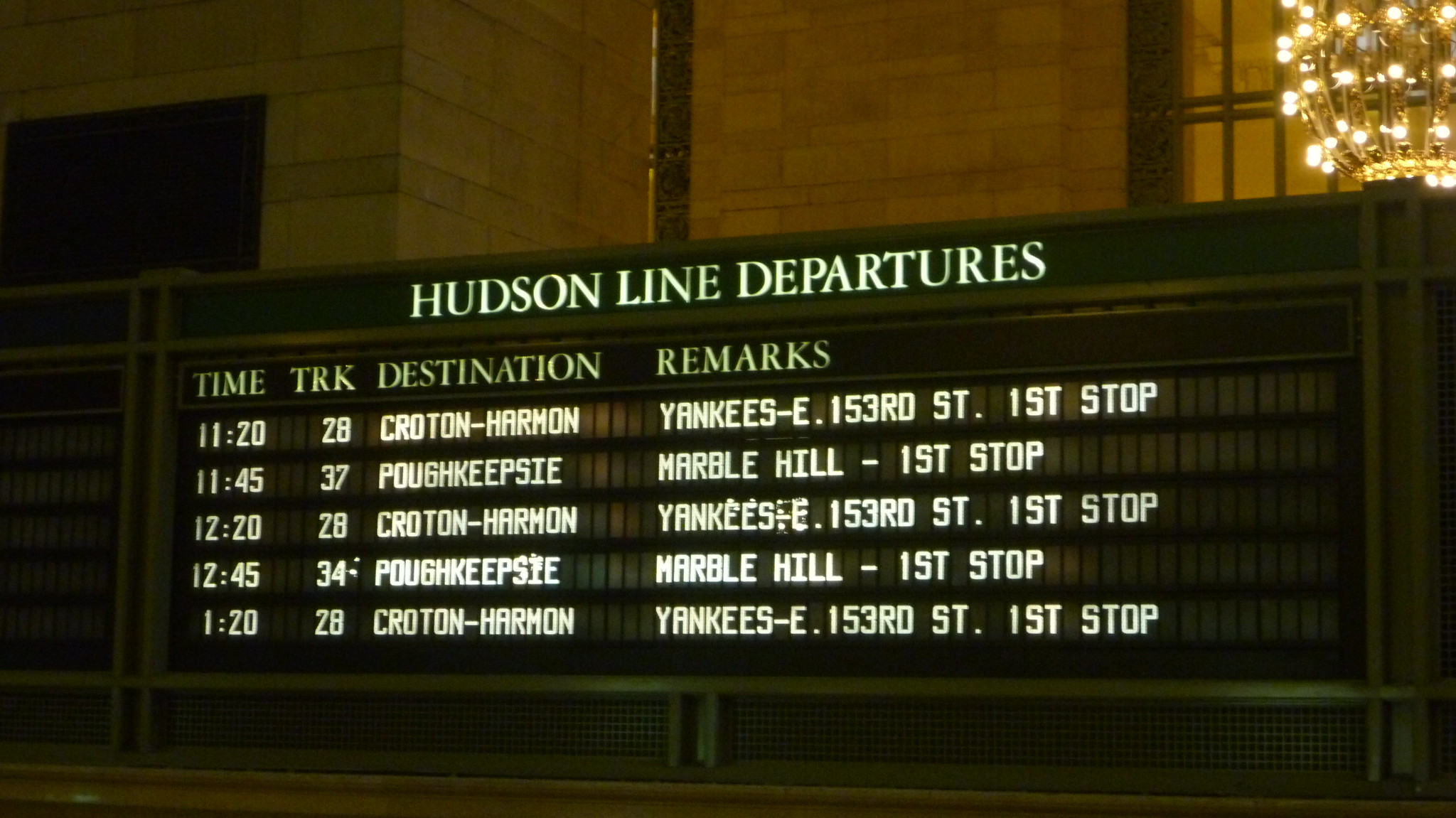In the image, there's a prominent departure board titled "Hudson Line Departures" featuring detailed information on train schedules. The board lists times, tracks, destinations, and remarks. Listed are: 11:20 on Track 28 to Croton-Harmon, with the first stop at Yankees East 153rd Street; 11:45 on Track 37 to Poughkeepsie, with the first stop at Marble Hill; 12:20 on Track 28, again to Croton-Harmon, with the first stop at Yankees East 153rd Street; and 12:45 on Track 34 to Poughkeepsie, with the first stop at Marble Hill. The sign indicates these are all Hudson Line departures. The departure board, taking up the central and lower portions of the image, is set against a backdrop of a stone wall. To the left, a darkness suggests the presence of a doorway. In the upper right corner, a lit chandelier with several bulbs is visible, enhancing the historical ambiance of the building.